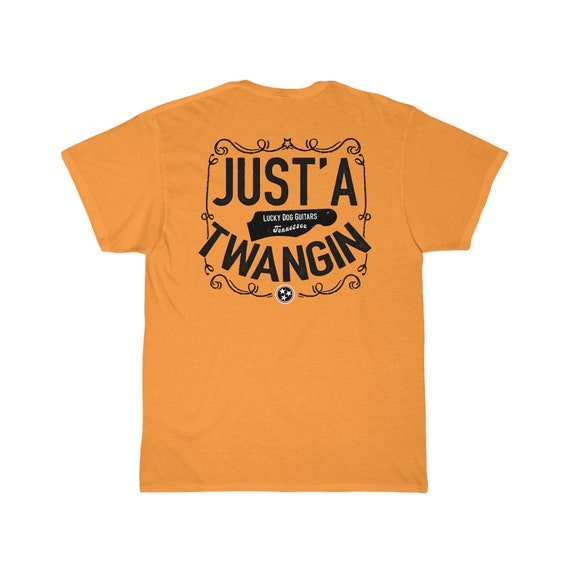This photograph features a vibrant orange short-sleeve T-shirt with a round neck, displayed against a clean, white backdrop. The T-shirt prominently showcases a central design composed of brown wavy lines forming a square frame. Within this frame, the text "JUST A' TWANGIN'" is written in all caps, with an apostrophe following "A." Centered between the words "JUST" and "TWANGIN'," there is a smaller black rectangular area that contains the white text "LUCKY DOG GUITARS" accompanied by an upper part of a guitar silhouette, with the word "TENNESSEE" written below it. Near the bottom of the design, a small circular emblem adorned with white stars highlights the detailed and artistic elements that encircle the central text. The overall layout includes vertical and curly patterns that add intricate detail to the T-shirt's design.